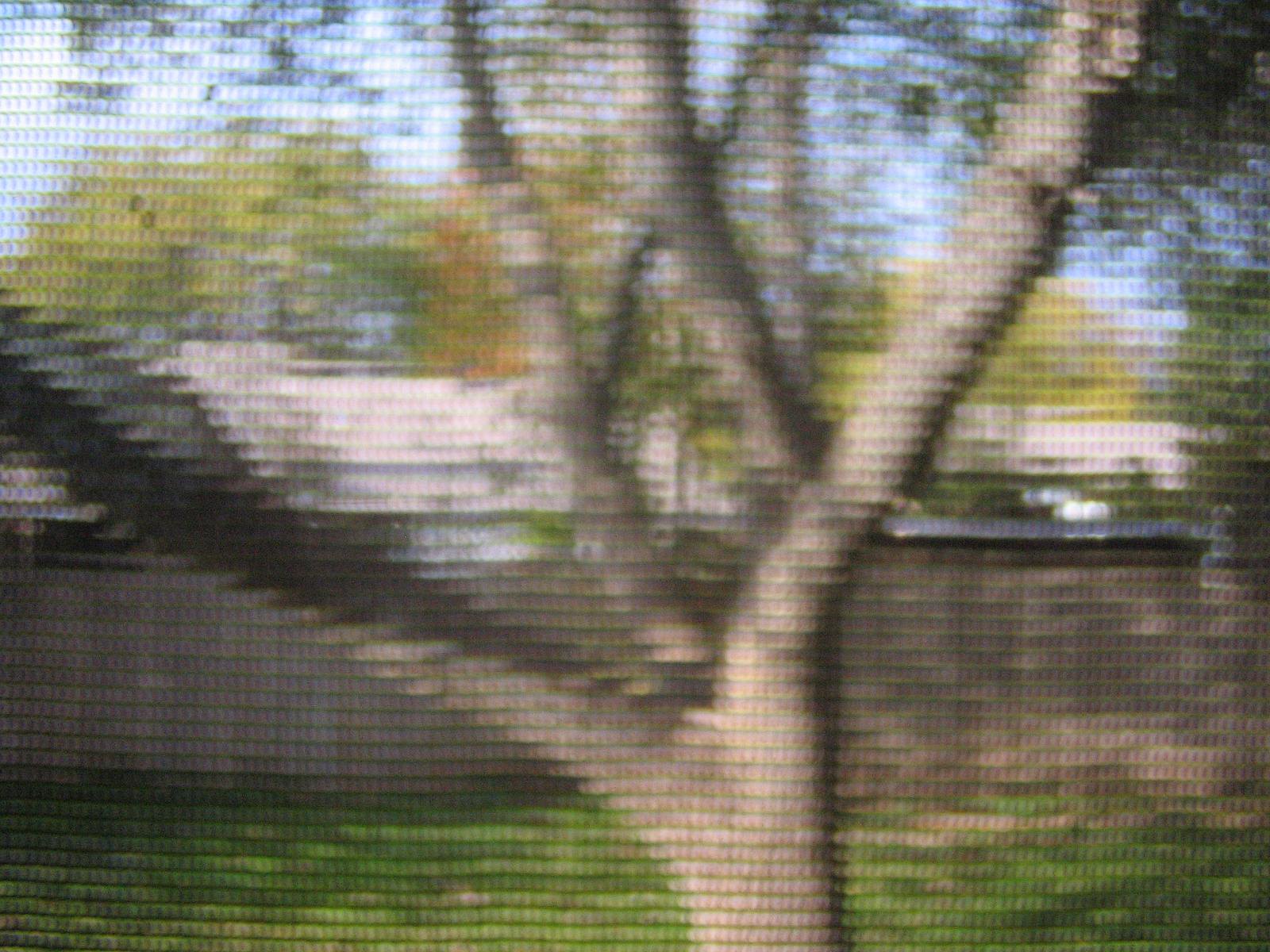The photograph captures a scene viewed through a window screen, resulting in a pixelated, grid-like overlay that blurs and obstructs the details. At the center is a large, branching tree trunk, surrounded by a lush green lawn. The bottom and top of the tree are not fully visible due to the cropping of the image. Behind the tree, there is a tall wooden privacy fence with a light blue sky peeking through above it. Beyond the fence, a white house stands partially obscured, with multiple mature trees boasting green and brown leaves in the background. The combination of the grid overlay from the window screen and the low, late afternoon light makes it challenging to discern finer details, rendering the entire image grainy and indistinct.